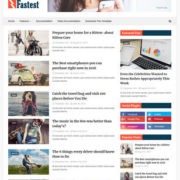This screenshot depicts a web page that appears to be either a blog or a news site. The overall quality of the image is poor, making the text and fonts difficult to discern.

In the upper left corner, there is what looks like the site name, "Fastest," written in black text. Next to the name is an orangish-red square featuring a white lightning bolt dividing the square into two sections.

To the right of this logo is a blurry, indecipherable photo. Below this, a light gray menu bar with five unreadable items spans across the page. The webpage's background is predominantly white.

On the left side of the page, a vertical column displays five blurry photos. The second photo appears to be a light green, old-style Volkswagen car. The third image looks like a close-up of a woman, though her face is not visible. The fourth image may show a woman seated in what seems to be a lounge chair. The bottom image features blue skies with white, fluffy clouds, green grass, and an indistinguishable figure.

At the center of the page, there are headlines and the first few sentences of several articles, though none are readable due to poor image quality.

On the right side of the page, a photo clearly shows a laptop displaying a colorful pie chart and graph. Below this image, in the sidebar section, are icons for social media platforms such as Twitter, Facebook, and Instagram.

At the bottom of the sidebar, three small, blurry photos are accompanied by unreadable headlines.